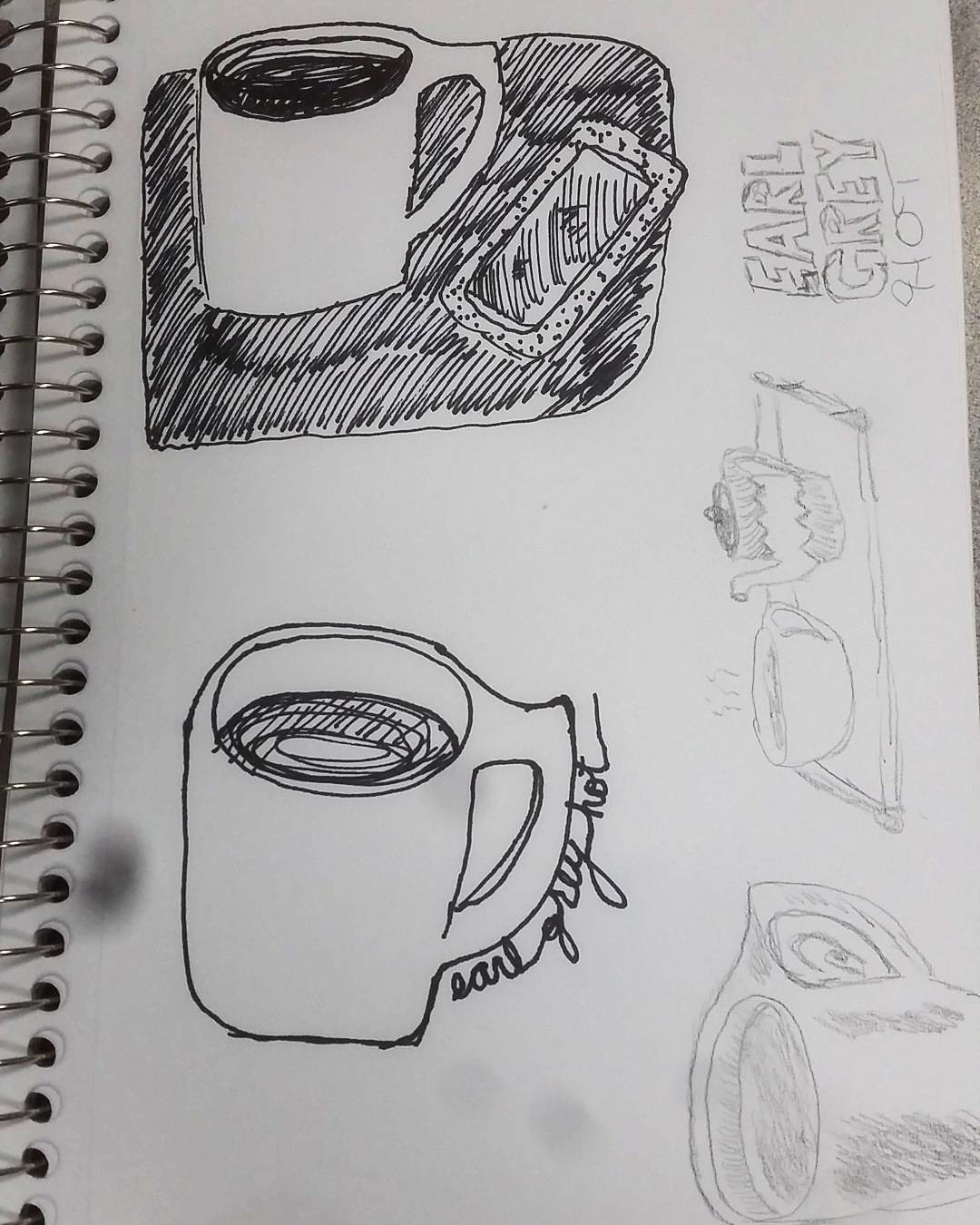A vertical photograph captures a sheet of white or off-white paper, likely in a spiral-bound sketchbook, as evidenced by a series of 30-40 hole punches and metal rings on the left side. The paper features multiple sketches primarily of cups and mugs, with careful details in various mediums. 

In the top left corner, there's a detailed pen ink drawing of a white mug filled with a dark liquid, situating on a black plate, accompanied by a smartphone tilted to the right. Below it, neatly rendered in black ink, is another white mug with dark liquid, bearing the cursive signature "Earl Grey Hot" along the handle, whose top slopes upward before extending straight back.

On the bottom left, a similarly sketched mug appears, also containing dark liquid. On the right side of the paper, sketches drawn in pencil dominate. One notable depiction, oriented 90 degrees counterclockwise, is a tray with a bowl and a kettle. Adjacent is a pencil-drawn inscription "EARL GREY" in bubble letters, and beneath it, "940T." The final sketch on the bottom right showcases another white mug with dark liquid, distinguished by grey brush strokes, adding texture and depth.

The sheet sits on a granite-like countertop, adding a subtle speckled beige and black background, indicating its placement and capturing the artistic process within a commonplace yet textured setting.